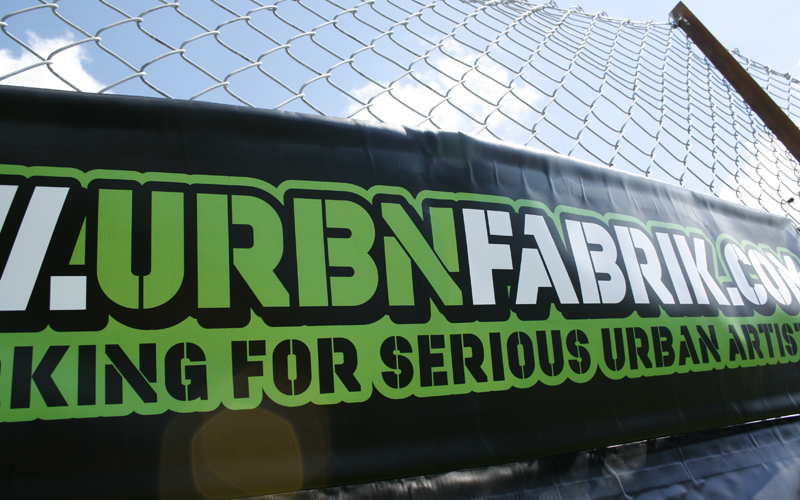The image depicts a close-up of a chain-link fence held up by a dark metal pole. Dominating about 90% of the picture, the fence is prominently featured against a background of a blue sky adorned with a few scattered clouds. Affixed to the lower middle section of the fence is a black plastic sign that partially advertises a website. The sign reads "urbnfabric.com" in white lettering, followed by "King for Serious Urban Artist" in green and black text. The sign appears to promote a website catering to urban artists. The contrast of colors—white and green on a black background—makes the text stand out vividly against the fence. The overall impression is of an advertisement likely placed in an outdoor space such as a stadium or other urban environment.